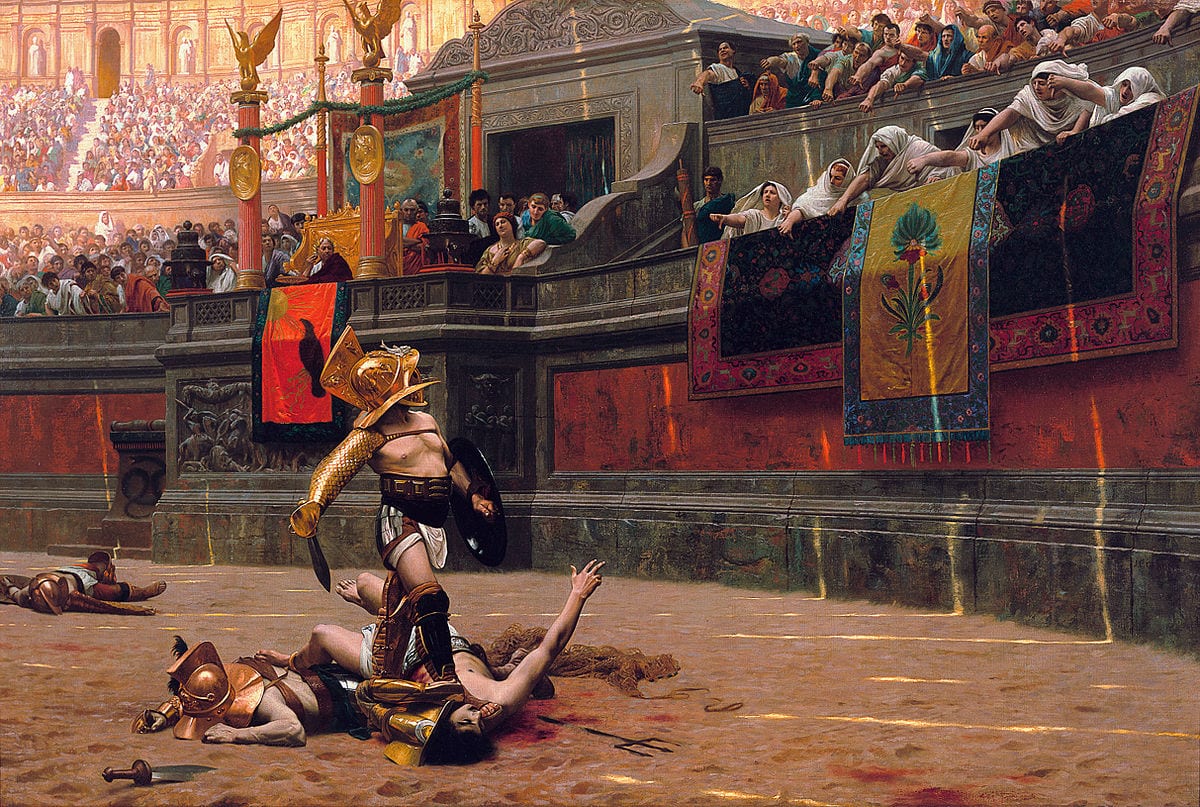The image is a highly intricate, horizontal rectangular drawing of an ancient Roman arena, depicting a brutal and chaotic blood sport. The scene is set on a dirt floor within an ornate, grand amphitheater made of dark gray granite blocks punctuated by red stripes. Dominating the arena are tall columns topped with golden birds with spread wings. Spectators fill the venue, arranged hierarchically with distinctions between the commoners and the more affluent.

At the front, women draped in white sheets hang over embroidered rugs—one blue with a yellow border and a central flower, the other black with a Victorian red floral pattern. They seem deeply engaged, heckling the combatants and showing gestures of disapproval, some with thumbs down. The combatants, resembling ancient gladiators, are in the midst of a fierce melee. One prominent figure, wearing a full-face gold helmet and minimal armor that exposes his chest, stands menacingly over a fallen opponent, a bloodied sword in his right hand and a black shield in his left. He appears triumphant but is met with mixed reactions from the crowd. Further in the background, another section of the audience is less hostile, perhaps indicating their support for the victorious gladiator. The overall composition suggests that this arena was a place of great spectacle and brutality, reflecting a time when human life was a mere entertainment.